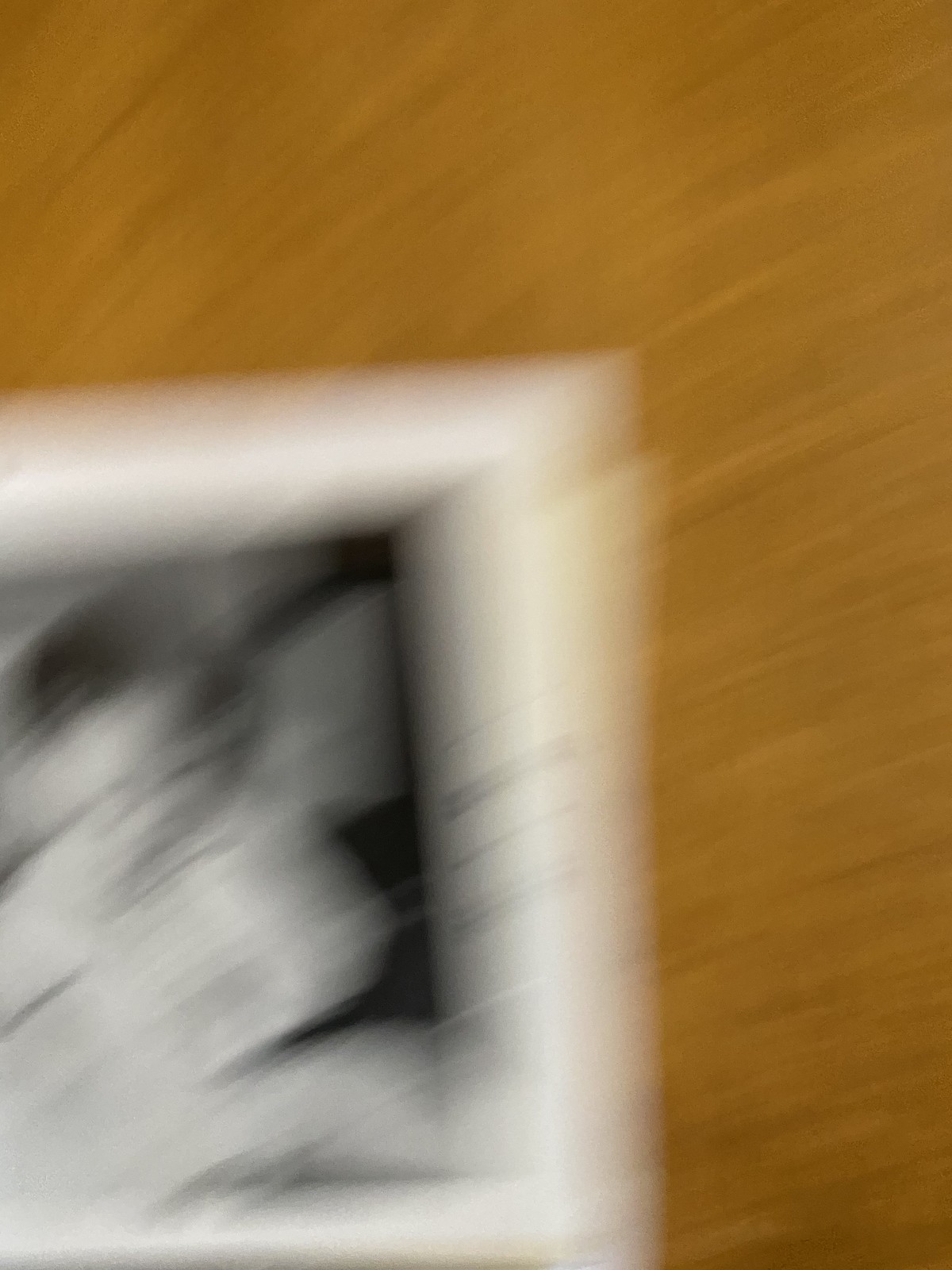This color photograph captures an extremely blurry image, making it challenging to discern whether it is an actual photograph or an illustration. The upper portion and the right-hand edge of the image showcase a light brown or tannish wooden background with a visible diagonal grain, suggesting it might be a wooden table. Positioned on this surface is a white picture frame with a black-and-white photograph inside. The image within the frame depicts a young child or baby who appears to be sitting down, with their right hand raised to their face. The child seems to be resting on someone, but due to the blurriness, this detail is difficult to confirm. Behind the child, the top part of the picture shows a grey area with a black shadow on the right-hand side. The entire scene is taken with such motion that every element, including the table, frame, and photograph, is rendered indistinct and fuzzy.